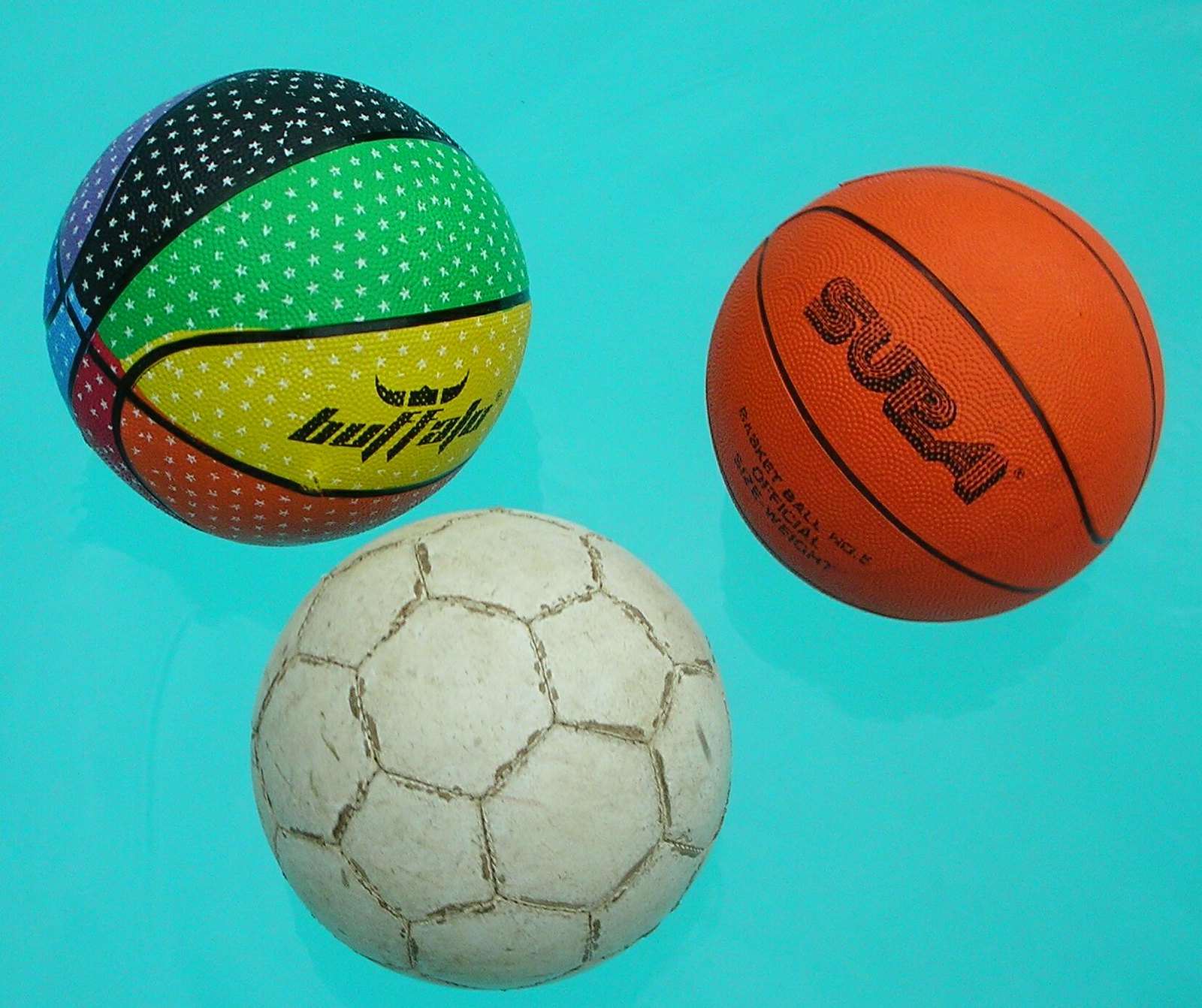This photo displays three sports balls against a light teal-blue background. The top left features a vibrant, multicolored basketball with sections in purple, dark navy, green, yellow, orange, red, and blue, all separated by black lines adorned with small white stars. The word "Buffalo" is emblazoned in black ink on the yellow section, with a set of horns. To the right, there is a traditional orange basketball marked with black lines. The brand name "Supa" (or "Sura") along with the phrase "Basketball Official Size and Weight" is visible, though some writings are unclear. In the bottom center, an all-white soccer ball with geometric hexagonal shapes, appearing well-worn with faded black markings, completes the trio of balls.